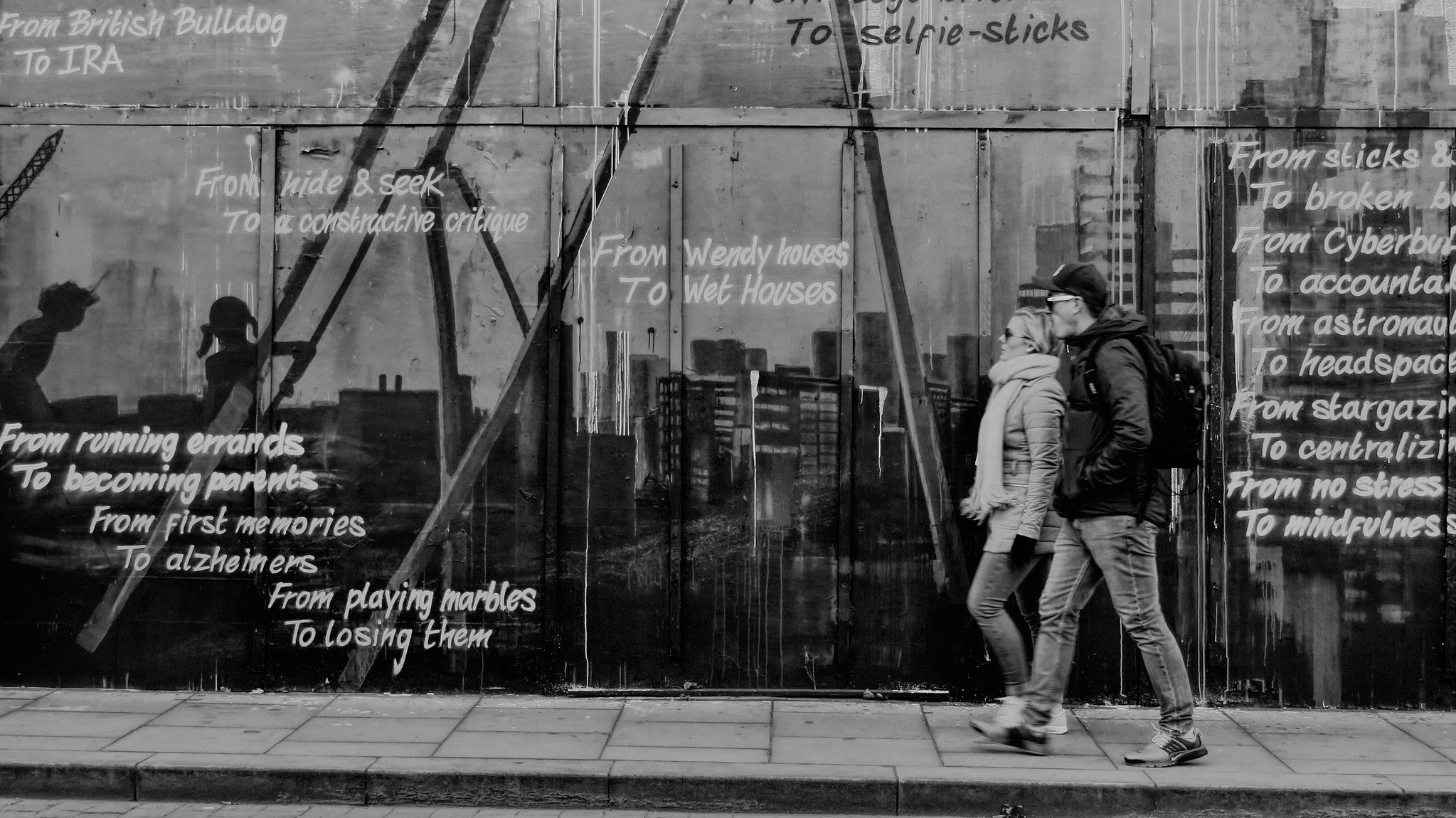This horizontally oriented, modern black-and-white photograph captures an outdoor city street scene. Two pedestrians, bundled up for the cold in down jackets, knitted scarves, jeans, and tennis shoes, walk along a sidewalk made of large blocks. The man is wearing a cap. They move in front of a building with a black plastic or glass facade adorned with wooden supports or slats, giving the impression of ongoing construction. 

Text is scattered throughout the image, including phrases like "From British Bulldog to IRA," "From Hide and Seek to a Coordinated Critique," and "From Running Errands to Becoming Parents." Other poignant lines, such as "From First Memories to Alzheimer's," "From Playing Marbles to Losing Them," and "From Sticks and Stones to Broken Bones," add layers of reflective poetry to the scene. Furthermore, phrases like "From Wendy Losers to Wet and Wet Houses" can also be found, contributing to the contemplative atmosphere.